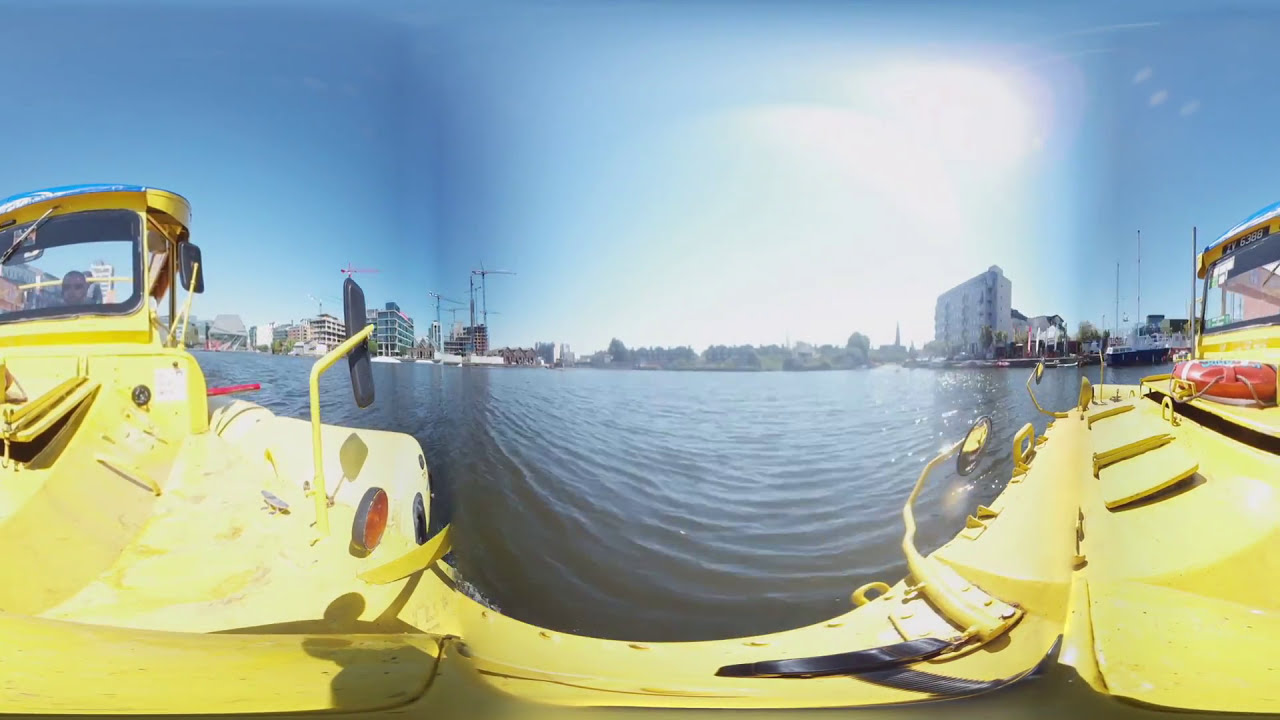The image, captured with a wide-angle lens from the center of a boat, showcases a vibrant canary-yellow, utility-style vessel on a dark, gently rippling body of water. The 360-degree perspective allows both ends of the boat to be visible, curving slightly due to the lens effect. A man with short, receding hair is seen in the cockpit, facing the camera. The background reveals a cityscape along the shoreline: to the left, numerous buildings and construction cranes; in the center, a stretch of greenery with bushes and trees; and to the right, a tall, distinct white building. Above, the clear blue sky is brightened by a blindingly radiant sun.